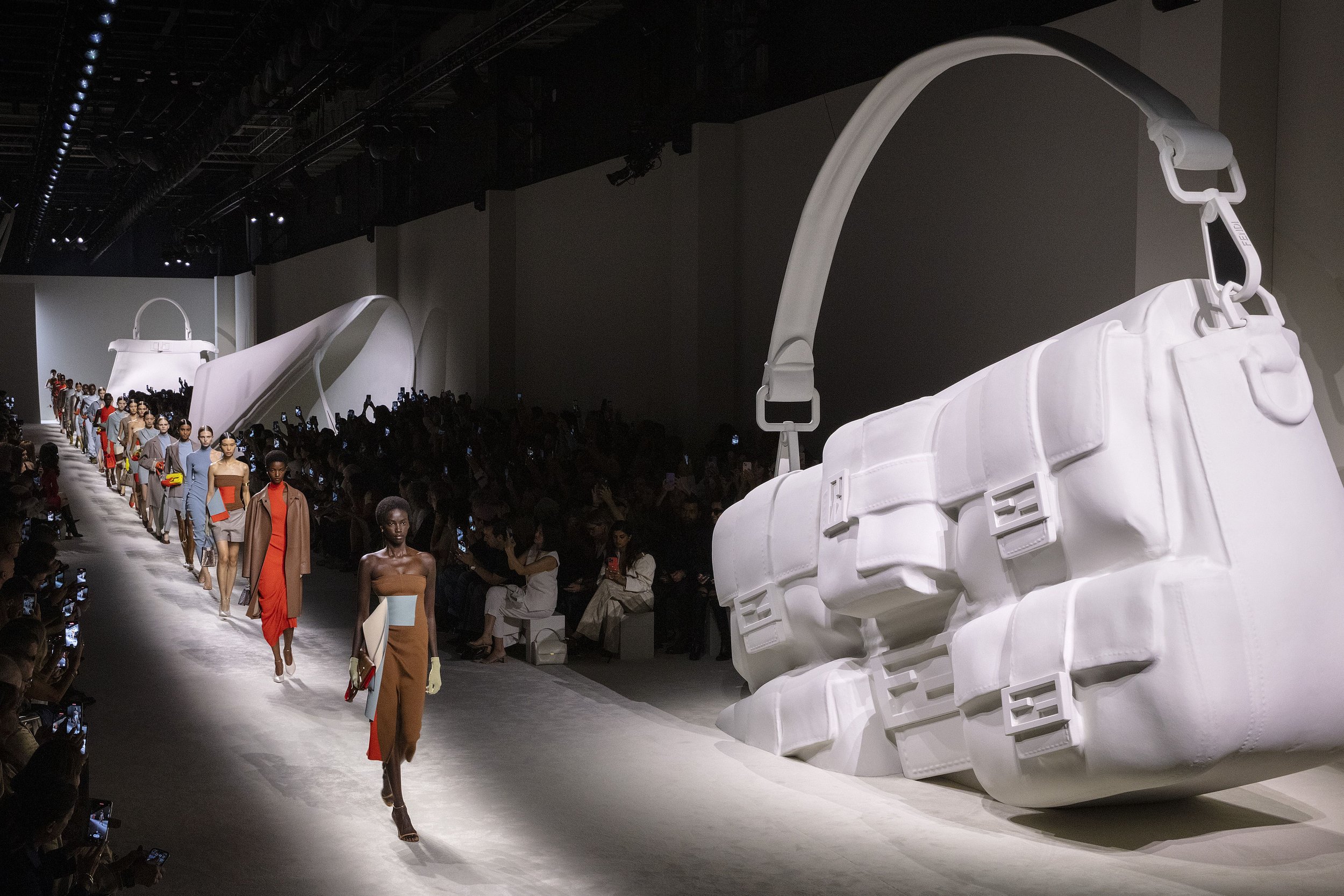The image is a detailed color photograph capturing a vibrant fashion show. On the right side of the image, prominently positioned from top to bottom, stands a colossal white purse with a gray strap, serving as an artistic centerpiece. To the left of this striking art piece is the runway, where a procession of around 25 models parades from the left foreground to the back middle of the image. The models, displaying a variety of outfits, walk in single file. The leading model, dressed in a brown outfit with a brown coat over a red dress, is followed by a diverse group of women: the first two are Black, the third appears Asian, the fourth White, and the fifth Indian, among others. Spectators flank both sides of the runway, seated and eagerly capturing the event with their phones, creating a sea of glowing screens. Three more giant, white artistic statues of purses, each estimated to be 15-20 feet tall, line the left side of the runway, enhancing the avant-garde atmosphere of the show. The image encapsulates the dynamic intersection of fashion, technology, and art.